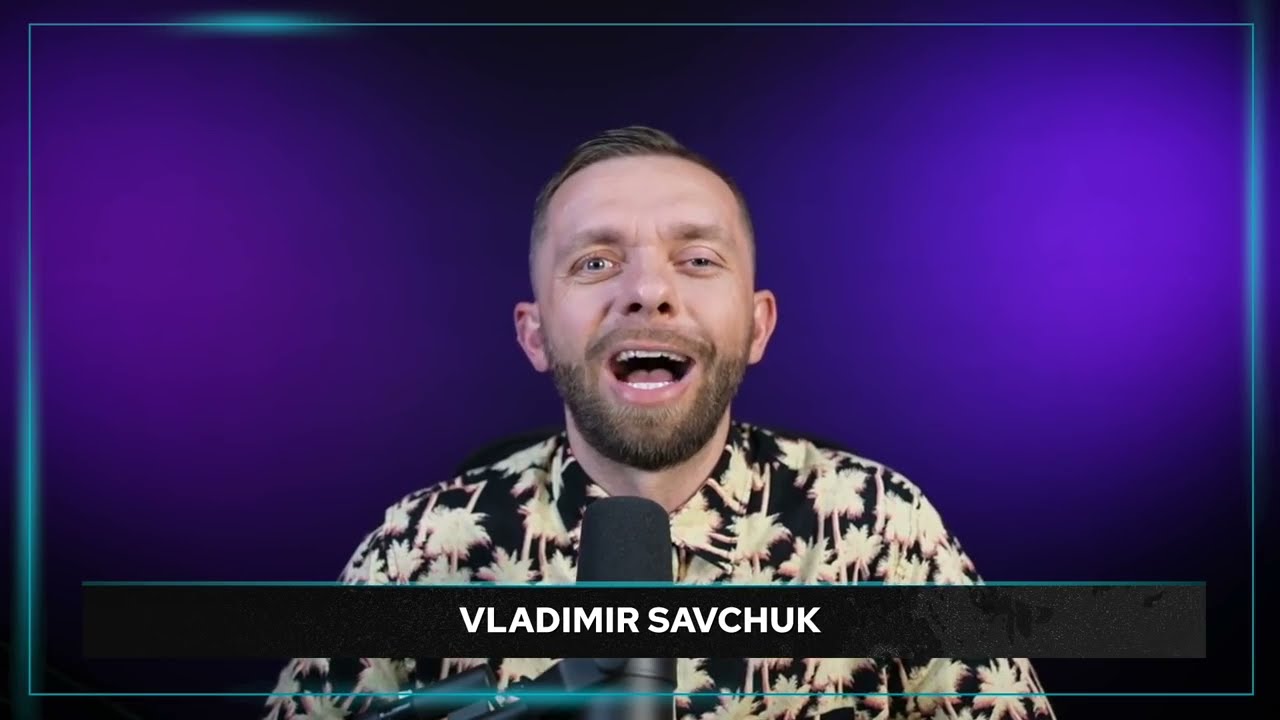The image features a white man with a brown beard, very short hair on top, and a lazy right eye that appears nearly closed. He is standing or sitting in front of a microphone, with his mouth open in a smile or laugh, looking directly ahead. He is dressed in a black button-down shirt adorned with yellow splotches resembling palm trees. The background is a purple gradient, darker on the left side and lighter on the right. Beneath him, there's a black bar with a teal line at the top, displaying his name in white font: "Vladimir Savchuk." Teal lines frame the image, adding an extra layer of design.